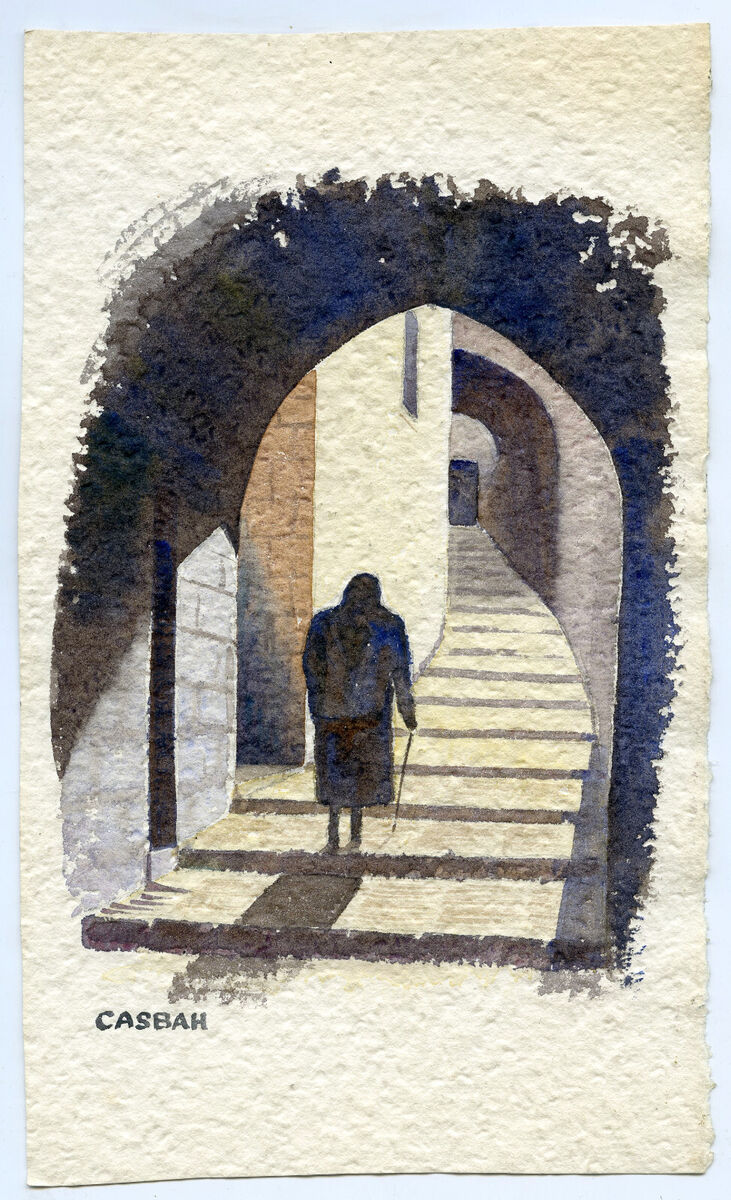This detailed illustration is rendered on a white, textured parchment with a tan hue, showcasing an evocative scene of an elderly woman walking through a stone hallway with a cane. The illustration features the woman, depicted in a dark, long coat, a dark skirt, and a head covering, as she ascends large rectangular stone steps. She is midway through the archways, which cast distinct shadow patterns. The stone walls of the hallway are marked by varying tones of white and brown, hinting at brick and stone textures. Above and around the woman, shadow details accentuate the windows, stairs, and the passageway. To her right are the stone buildings, and a stone door lies at the far end of the tunnel-like alleyway. At the bottom left corner of the artwork, the name CASBAH is inscribed in dark ink, signifying the artist’s signature. The scene’s intricate details are enhanced by the lighting which possibly includes dark leaves or additional shadows, enriching the atmospheric depth of this simplistic yet deeply textured drawing.